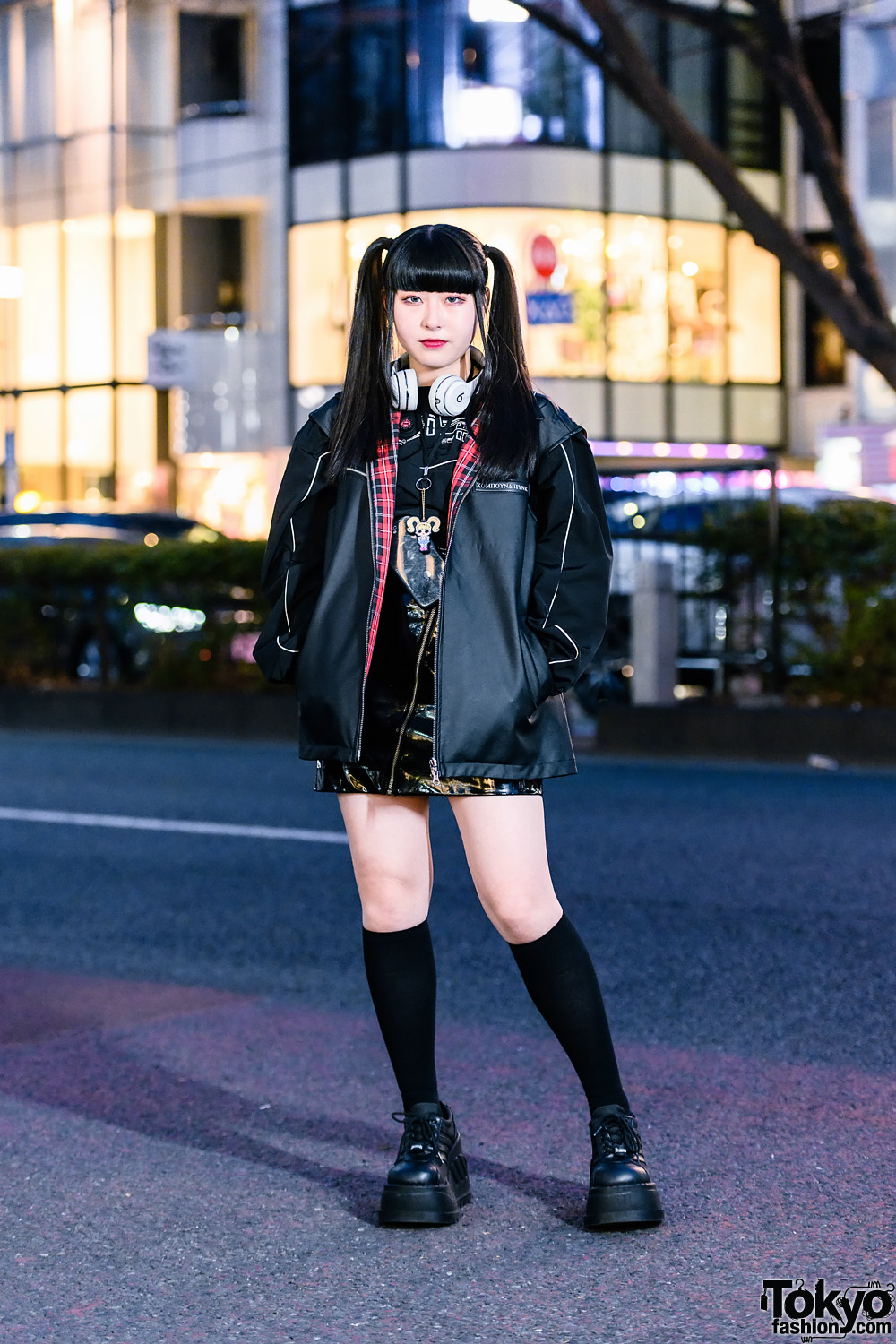This photograph features a young Asian woman in her early 20s standing confidently on a street in Tokyo at night, as indicated by the "TokyoFashion.com" watermark in the lower right corner. The background displays a softly blurred image of a building and a car, with the dark asphalt underfoot. She exudes a trendy, hipster vibe, dressed in a striking black and yellow short dress adorned with multiple zippers. Over the dress, she sports an open, long-sleeved black leather jacket, lined with a bold red, white, and black plaid pattern. The jacket features a prominent white stripe down the middle and her hands rest casually in its pockets. She accessorizes with knee-high black socks and chunky, male-styled black shoes that resemble combat boots. Her straight, brunette hair is styled in two side ponytails with blunt bangs framing her face. She wears a hint of red lipstick and has white headphones draped around her neck, adding a touch of modern flair to her look. A small owl detail decorates her black shirt, adding a whimsical touch to her fashionable ensemble. Staring directly into the camera with a serious expression, she is a compelling presence in this street fashion scene.